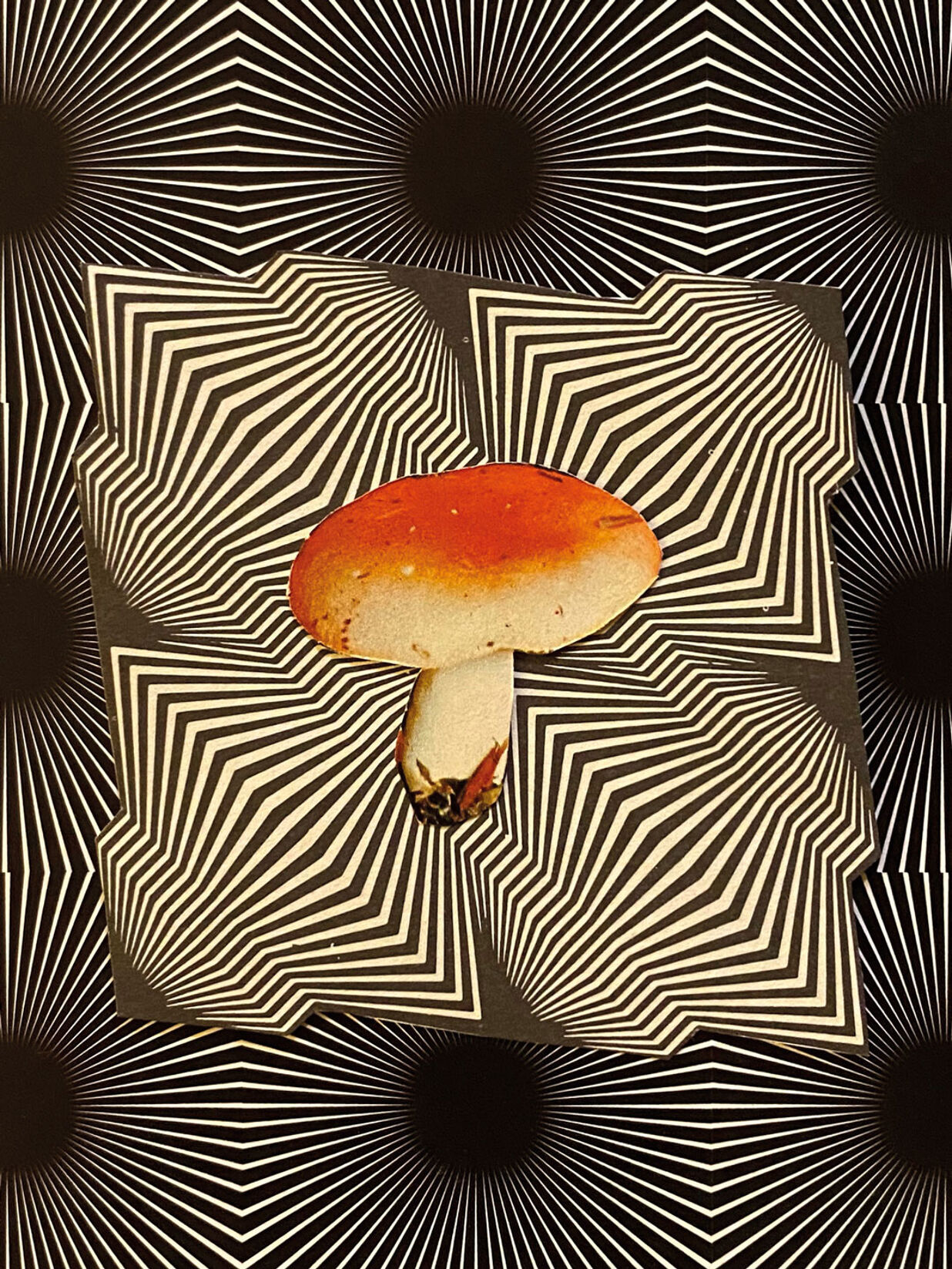In the center of this digital artwork is a striking photograph of a mushroom. The mushroom features a large, bread-colored cap with hues of beige and orange, perched atop a somewhat off-white, yellowish stalk. At the base, hints of dark brown elements, possibly sticks and dirt, can be seen. The mushroom stands in sharp contrast to the intricate background, composed of repeated black and white geometric patterns. These patterns form an optical illusion, with fine lines creating a sense of movement and shifting perspectives. The background features a grid of four identical squares, each containing a feathered black circle at its core, from which thin lines radiate outward. This design element enhances the psychedelic feel of the artwork, suggesting a surreal, almost hypnotic visual experience.